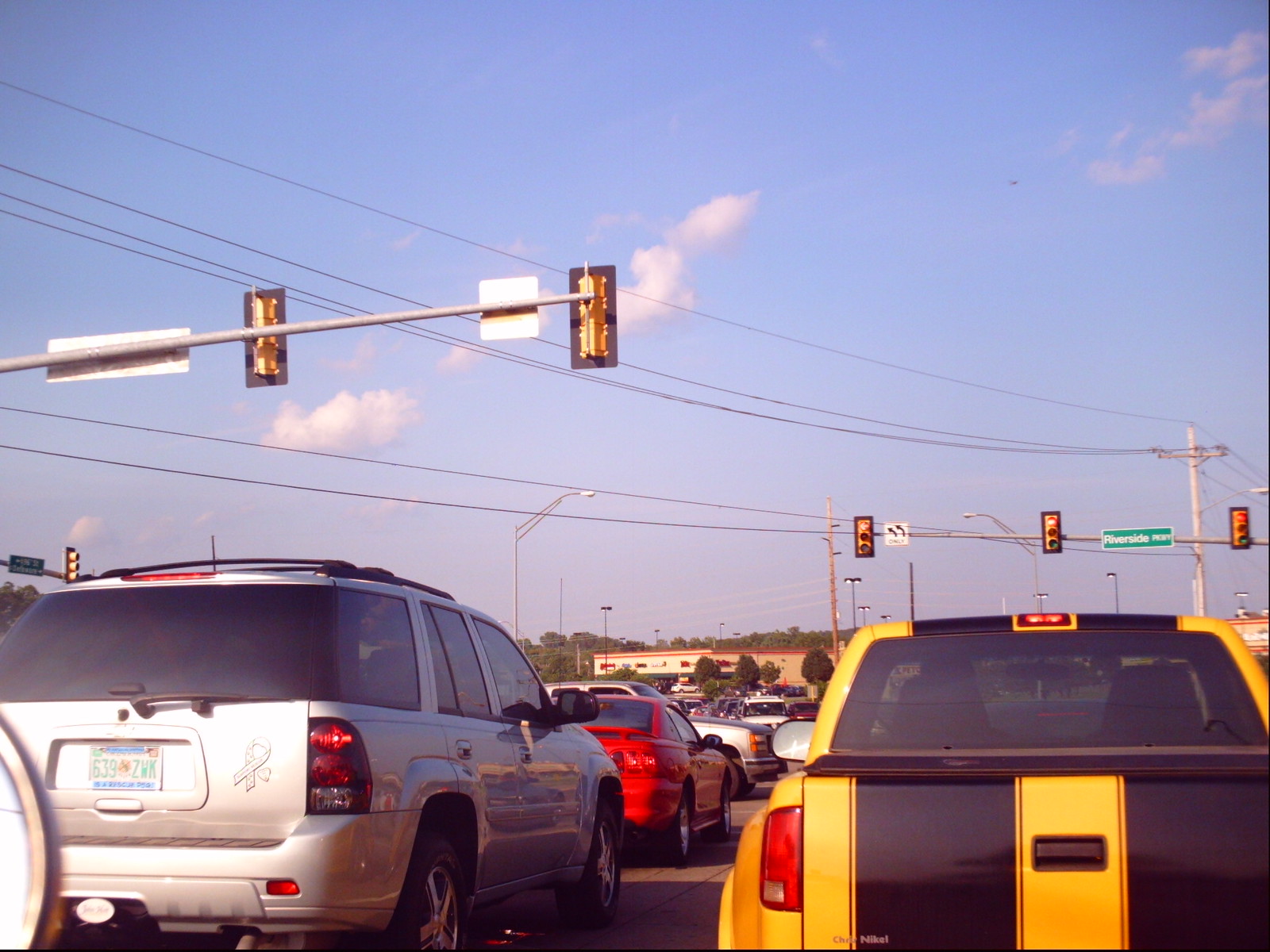This photograph captures a bustling intersection on a bright, sunny day, characterized by clear, blue skies interspersed with a few fluffy white clouds. Dominating the midsection of the image are black power lines strung between sturdy wooden poles. Prominently featured in the center are the sleek, silver arms holding multiple traffic lights. Two of these traffic lights face away from the viewer, while three lights, directed towards the viewer, display a vivid red signal. 

In the lower part of the photograph, a variety of vehicles are queued up. Notably, there's a distinct yellow truck with bold black stripes, a gleaming silver SUV, and a classic red sedan. Adding to the scene's dynamism, a truck is seen crossing the intersection perpendicularly to the halted traffic. The image vividly portrays a typical scene at a busy roadway intersection under the clear afternoon sky.